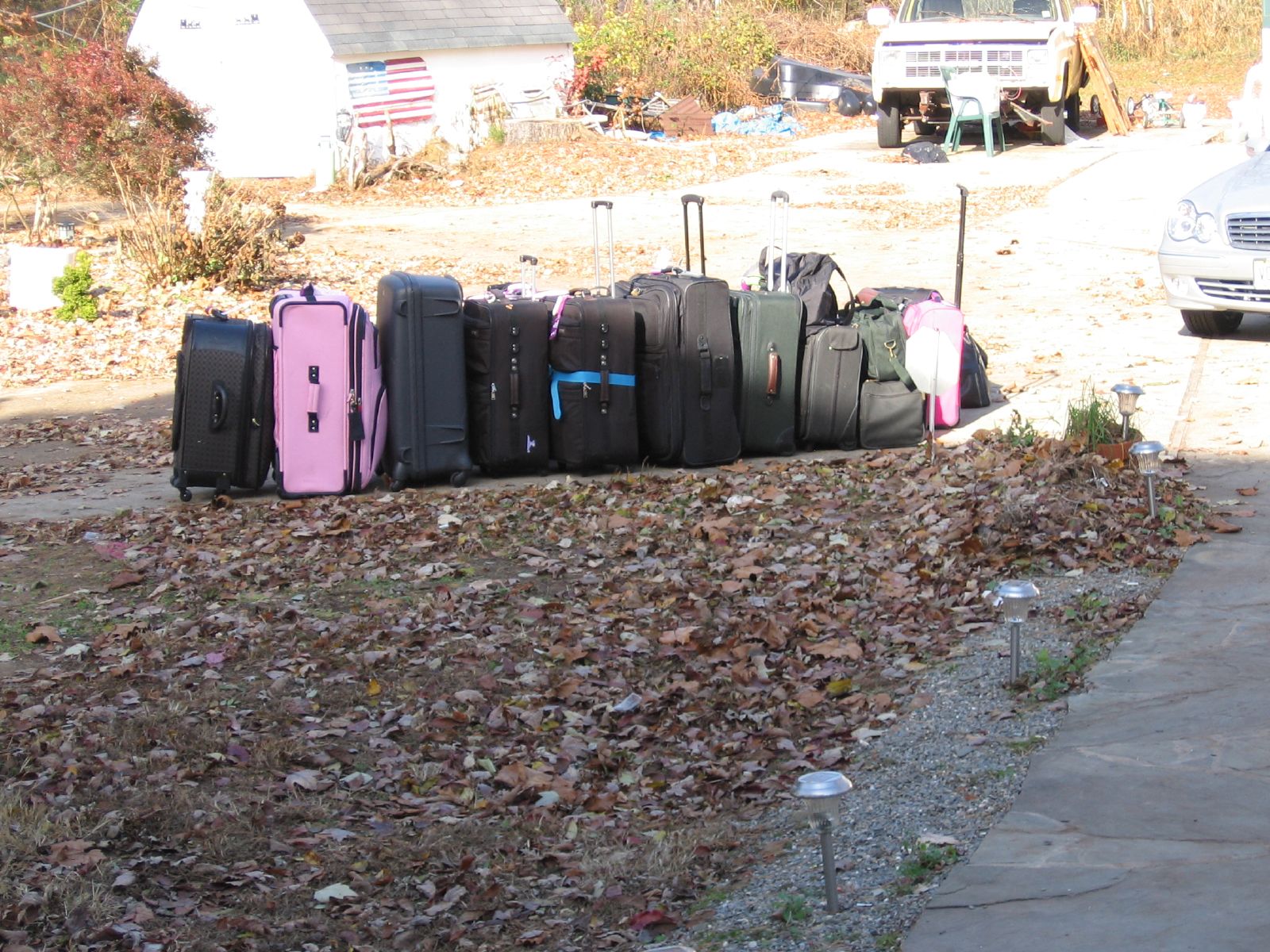The image depicts a cluttered outdoor scene, possibly someone's backyard or driveway, covered in autumn leaves. Central to the picture is a line of assorted luggage—around twelve pieces in total—ranging in size, color, and style. Among the suitcases, there are hot pink, classic black, navy green, and even a few duffel bags, representing a mix of hard plastic and cloth materials. This array of luggage stretches from the bottom right corner of the image and extends to the right, beside a brick walkway with adjacent gravel, and a few spaced-out silver lights.

In the upper center-right part of the photo, the front end of a silver sedan with two headlights is visible. To the right, there is another concrete walkway lined with the luggage. Prominent pieces include a small black bag resting on a green suitcase, a longer black bag, two identical-sized black suitcases, a brown and green stacked suitcase, and a distinctive white and pink suitcase with an extended handle.

The background showcases a mix of natural and man-made elements. A tree, painted with fall colors of brown and green, spans the top left edge. Directly behind the luggage line is a white shed adorned with an American flag, its roof covered in gray shingles, bathed in afternoon sunlight. More brown and green trees frame the right side of the image. Further to the right, a white truck with its hood slightly open and what appears to be slabs of wood hanging from it, sits idle. This truck appears out of service, adding to the scene's neglected ambiance. Leaves blanket the ground thickly, suggesting a fall season setting.